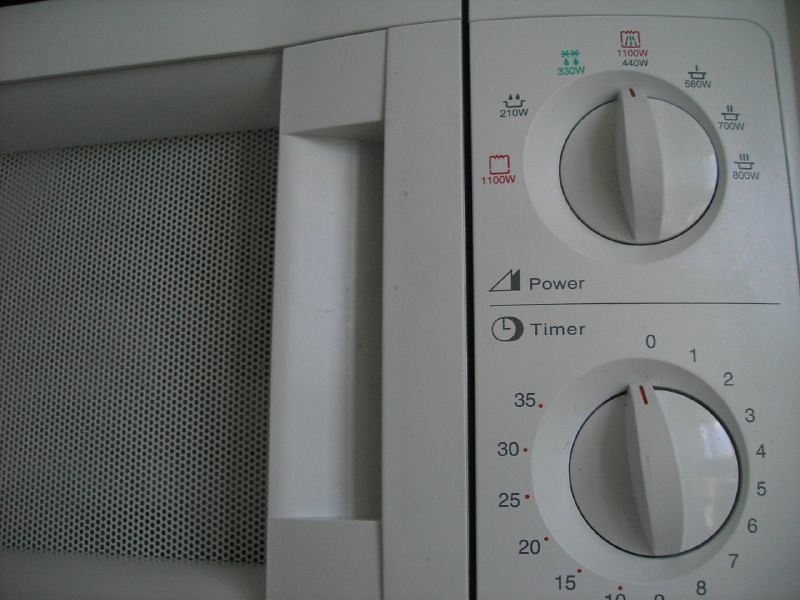This image is a detailed, up-close photograph of a white plastic microwave, primarily showcasing its control knobs on the right side of the appliance. In the center of the frame is the microwave door handle with a partial view of the frosted glass front. The photograph, though dimly lit and not well-cropped, clearly depicts two main control dials. The top dial, labeled "Power," features multiple wattage settings arranged in a semicircle, including 1100 watt (red), 210 watt (black), 330 watt (green), 1100 watt (red), 440 watt (black), 580 watt (black), 700 watt (black), and 800 watt (black). This power dial is currently set between 1100 and 440 watts. The lower dial, labeled "Timer" with a clock symbol next to it, sets the cooking duration from 0 to 35 minutes, with intervals marked at every 5 minutes. Both dials are white with clear labels. The overall scene suggests an everyday, functional kitchen appliance with a simple design.